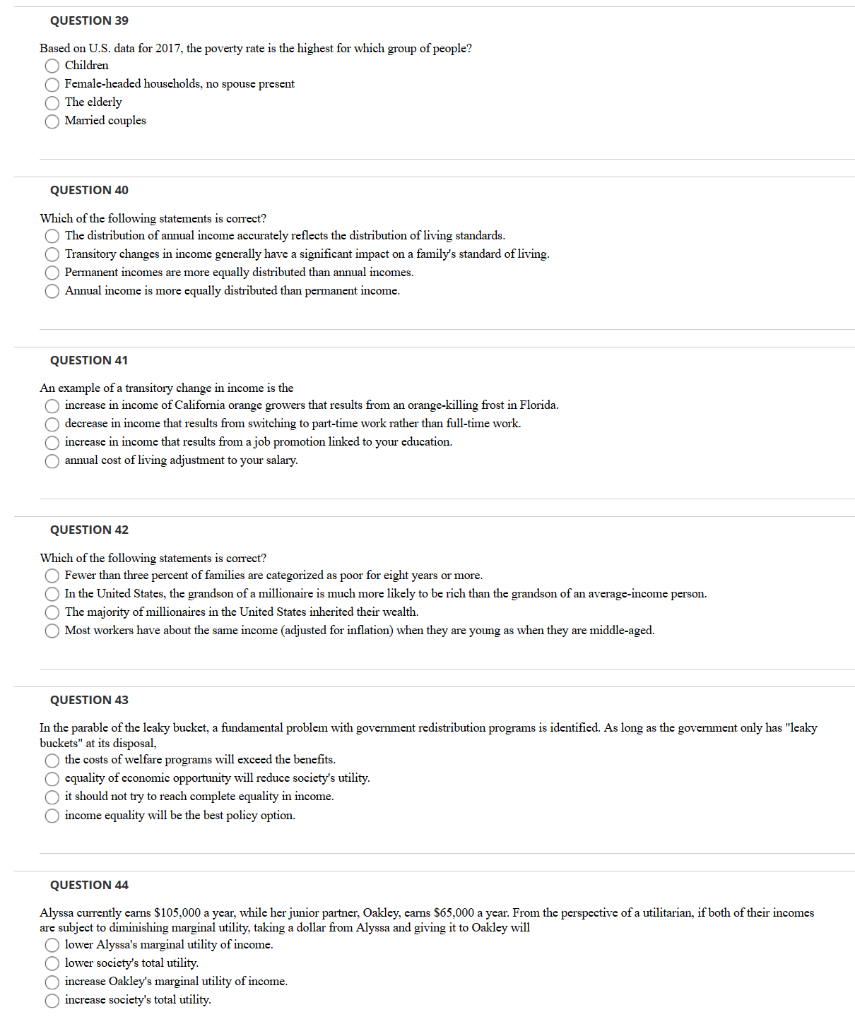This image captures a detailed view of a quiz or survey presented on a digital screen, comprising six multiple-choice questions. Each question is contained within individual blocks, with clear formatting that includes thick black lettering for the question numbers and main text, followed by options in smaller, thinner lettering, each accompanied by checkboxes for responses.

**Question 39:**
In bold text, "Question 39," followed by:
"Based on US data for 2017, the poverty rate is the highest for which group of people?" 
The available options are:
- Children
- Female-headed households with no spouse present
- The elderly
- Married couples

**Question 40:**
In bold text, "Question 40," followed by:
"Which of the following statements is correct?"
The available options are:
- The distribution of annual income accurately reflects the distribution of living standards.
- Transitory changes in income generally have a significant impact on a family's standard of living.
- Permanent incomes are more equally distributed than annual incomes.
- Annual income is more equally distributed than permanent income.

**Question 41:**
In bold text, "Question 41," followed by:
"An example of a transitory change in income is:"
The available options are:
- The increase in income of California orange growers that results from an orange-killing frost in Florida.
- Decrease in income that results from switching to part-time work rather than full-time work.
- Increase in income that results from a job promotion linked to your education.
- Annual cost of living adjustment to your salary.

**Question 42:**
In bold text, "Question 42," followed by:
"Which of the following statements is correct?"
The available options are:
- Fewer than three percent of families are categorized as poor for eight years or more.
- In the United States, the grandson of a millionaire is much more likely to be rich than the grandson of an average-income person.
- The majority of millionaires in the United States inherited their wealth.
- Most workers have about the same income adjusted for inflation when they are young as when they're middle-aged.

**Question 43:**
In bold text, "Question 43," followed by:
"In the parable of the leaky bucket, a fundamental problem with government redistribution programs is identified. As long as the government only has leaky buckets at its disposal:"
The available options are:
- The costs of welfare programs will exceed the benefits.
- Equality of economic opportunity will reduce society's utility.
- It should not try to reach complete equality in income.
- Income equality will be the best policy option.

**Question 44:**
In bold text, "Question 44," followed by:
"Alyssa currently earns $105,000 a year, while her junior partner Oakley earns $65,000 a year. From the perspective of a utilitarian, if both of their incomes are subject to diminishing marginal utility, taking a dollar from Alyssa and giving it to Oakley will:"
The available options are:
- Lower Alyssa's marginal utility of income.
- Lower society's total utility.
- Increase Oakley's marginal utility of income.
- Increase society's total utility.

Each of these questions is accompanied by possible answers, set beside individual checkboxes for selection, making the format clear and user-friendly. The questions appear to be focused on economic concepts and social statistics, likely sourced from a textbook or online educational resource.